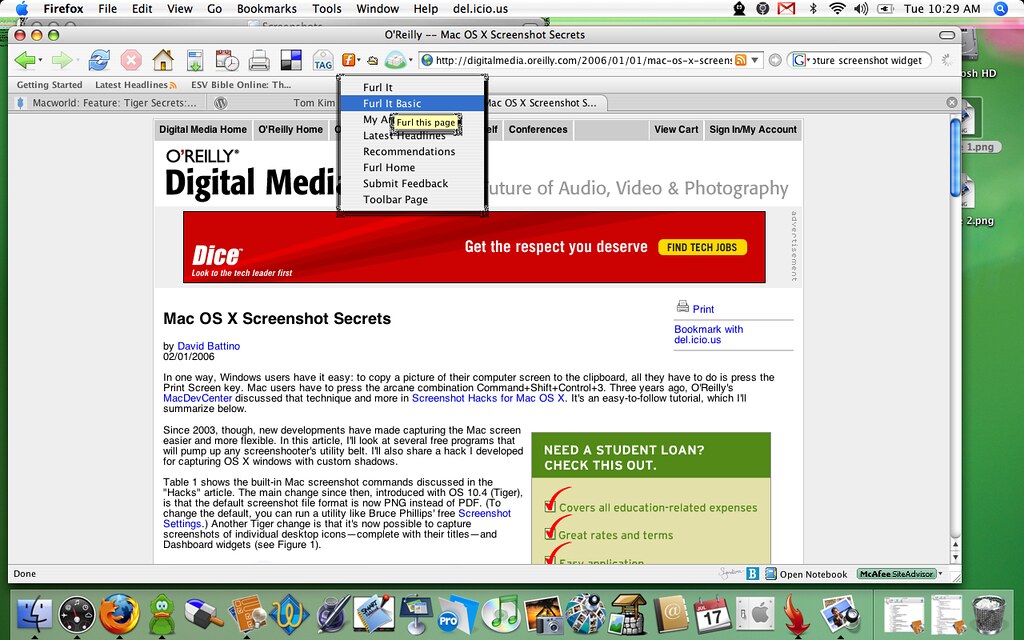The image captures a screenshot of a mid-2000s Mac OS desktop. The desktop displays a selection of application icons at the bottom, including Finder, Safari, and Firefox. Open in the old Firefox browser is a webpage from O'Reilly Digital Media that discusses the future of audio, video, and photography. Prominently featured on the webpage is an article titled "Mac OS X Screenshot Secrets" authored by Daniel Bortino, dated 0201-2006. The browser window shows a menu dropdown from an extension named FURL, with options like FURL It, FURL It Basic, My Account, Latest Headlines, Recommendations, FURL Home, Submit Feedback, and Toolbar Page. The overall display reveals the typical old-style icons and the layout of an older Mac OS, complete with a white top menu bar. Additionally, there is an advertisement on the page for Dice, promoting tech job opportunities with the tagline "Get your respect you deserve."